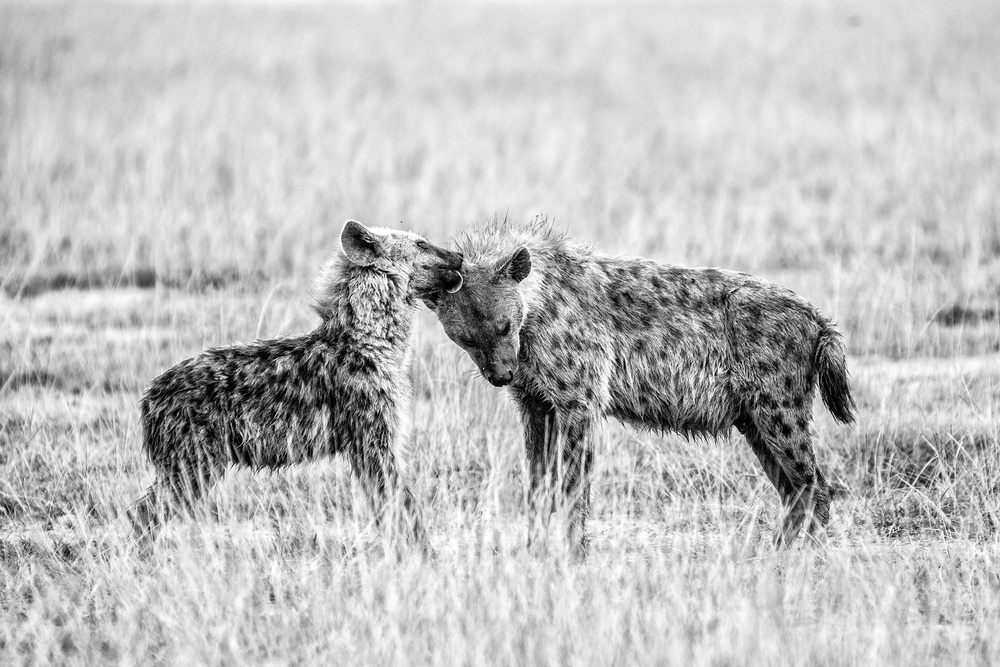In this striking black and white wildlife photograph, set in a natural environment, two hyenas are captured standing in a wide field of medium-height grass that reaches up to their bodies. The central focus of the image is on the interaction between the two hyenas: the slightly smaller hyena on the left has its head raised and is lovingly licking the forehead of the larger hyena on the right, whose head is lowered towards the ground. The hyenas, both furry and covered in distinctive black spots, exhibit a slightly disheveled appearance. Their short tails and curved ears are also visible, with the tail of the larger hyena appearing lighter on the top and darker on the bottom. The shot is framed horizontally, emphasizing the intimate moment between the animals amidst the natural backdrop.